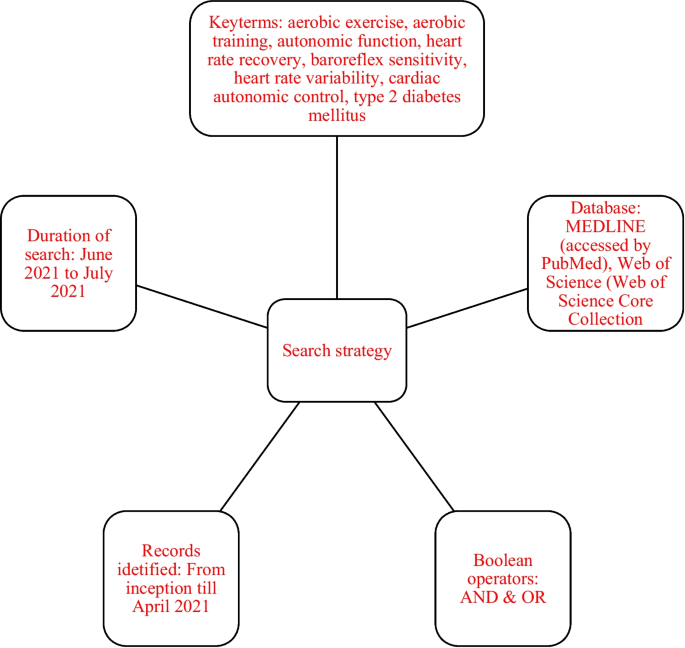The image features a star-shaped flowchart set against a white background, with a central black-outlined rectangle labeled "Search Strategy" in red typewriter font. Five black lines radiate outward in a sunburst pattern, each connecting to a black-bordered box with details in red text. The top box is labeled "Key Terms" and lists aerobic exercise, aerobic training, autonomic function, heart rate recovery, baroreflex sensitivity, heart rate variability, cardiac autonomic control, and type 2 diabetes mellitus. To the upper right, the box labeled "Database" mentions MEDLINE (accessed by PubMed) and Web of Science (Core Collection). Moving downward to the lower right, the box details "Boolean Operators" with "AND" and "OR" in all caps. The lower left contains a box labeled "Records Identified" from inception till April 2021. Lastly, the upper left box specifies the "Duration of Search" from June 2021 to July 2021. This detailed diagram is entirely monochromatic except for the vivid red text inside the outlined boxes.